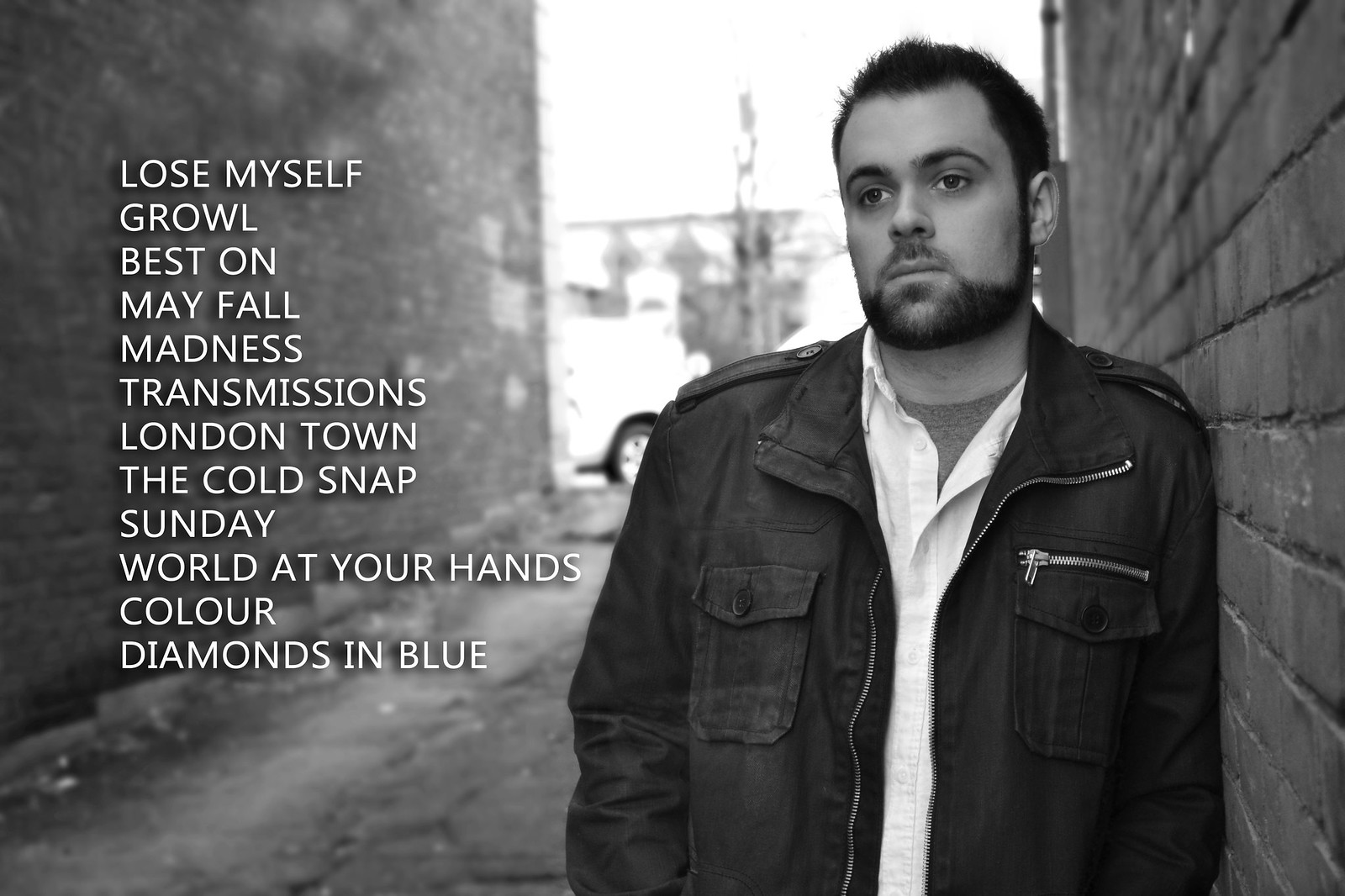A black-and-white landscape photograph captures a man standing in an alleyway, leaning casually against a brick wall on his right. The subject, a bearded man in his mid-thirties with short black hair, wears a black, open zip-front jacket over a white shirt and a gray undershirt. His expression is vacant, and he gazes downwards to the left, appearing somewhat disconnected. The alleyway, illuminated by daylight, has several cars in the background, suggesting a busy urban setting. To the left of the man, a column of white text is aligned vertically, possibly listing song titles: "Lose Myself, Growl, Best On, May Fall, Madness, Transmissions, London Town, The Cold Snap, Sunday, World at Your Hands, Color, Diamonds in Blue." This carefully framed composition, with its realistic representation and use of typography, evokes a sense of contemplative isolation, possibly hinting at an album cover's artistic intent.